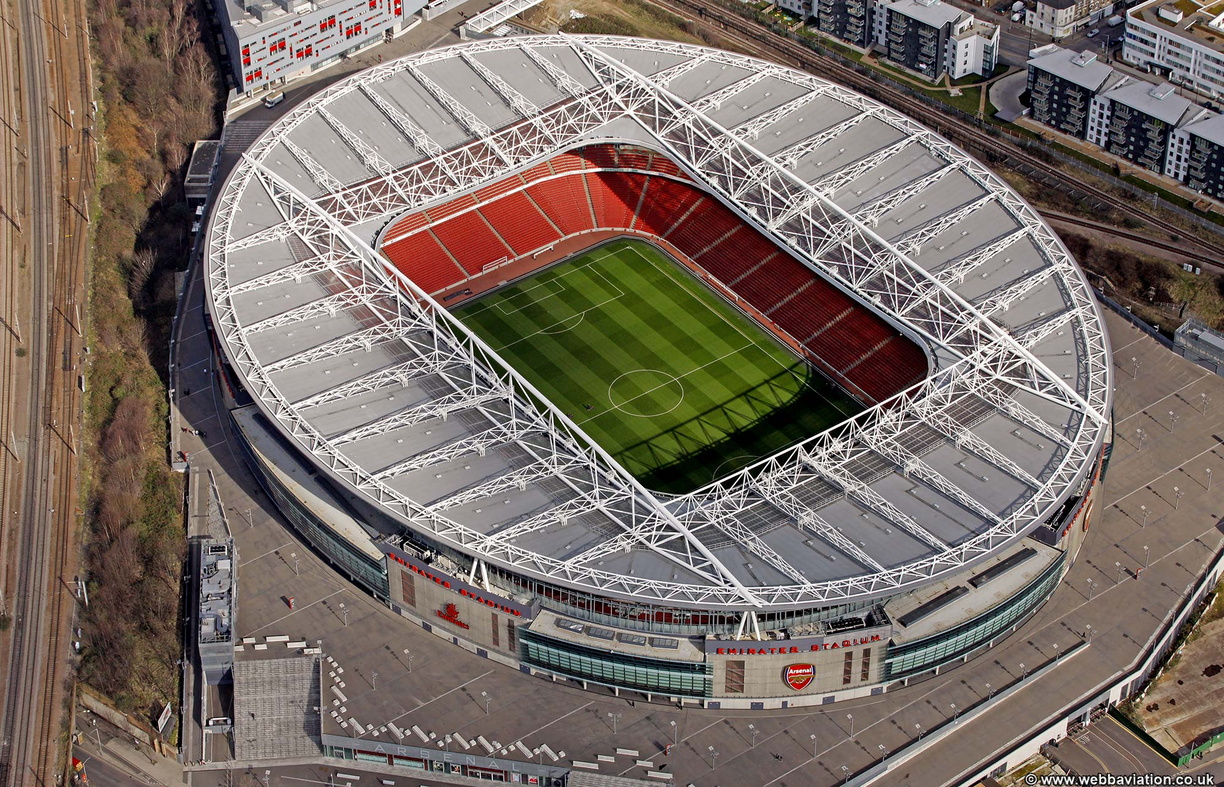This is an aerial view of the Emirates Stadium in England, capturing its intricate design and surrounding area in great detail. The stadium, primarily used for soccer, features an oval shape with a silver roof adorned with white metal beams that create a rectangular opening in the middle. Through this opening, you can see the pristine green grass of the field, meticulously patterned with light and dark green stripes, and the white playing lines. The seating encircling the field is uniformly red.

Over the entrance, there's a display with red letters spelling out the stadium's name, above a red insignia, though it's hard to decipher the exact text. The image also shows various entry points and possible ticketing offices with windows near the stadium's lower parts. The exterior of the stadium is complemented by surrounding apartment buildings with red-trimmed windows and further accentuated by vegetation consisting of green and brown greenery neatly planted near a visible railroad track on the left.

The stadium holds a dominant place in the photograph, implying its substantial size, with roads, additional buildings, and parking areas appearing on the outer edges, especially toward the right and left sides of the image. The well-planned environment of Emirates Stadium is a testament to its significance and modern architectural beauty.